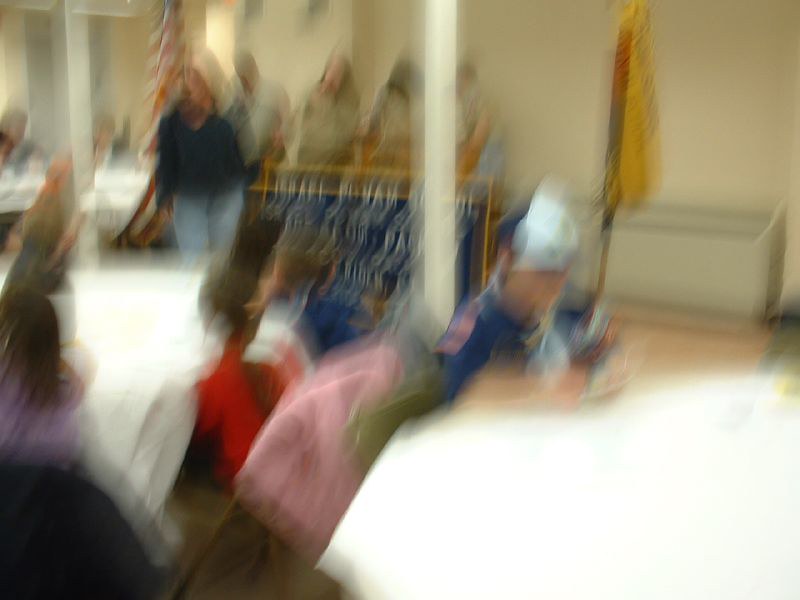The image is of low resolution and is quite blurry, making the details hard to discern. It has a square shape and features a group of people, some standing in the background and others seated in the foreground. An American flag is visible in the top left corner, positioned behind one of the standing individuals. On the top right, there is another flag, which is yellow in color, hanging against a white wall. A table is located in the bottom right corner of the image.